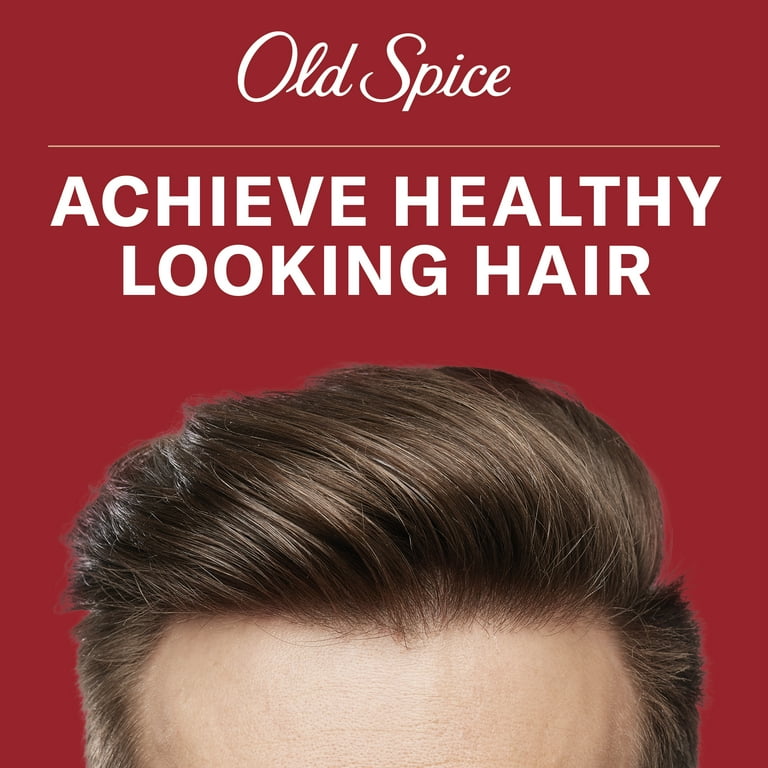This Old Spice ad features a deep red background with the classic Old Spice script prominently at the top. Below the script is a thin white line, and beneath the line, in bold, all-caps sans serif font, are the words "Achieve Healthy Looking Hair." The lower half of the ad showcases the top part of a man's head and forehead. His healthy-looking, well-groomed light brown hair is parted on the right and combed over to the left, with the top section brushed back and shiny under a light source coming from the left. The sides of his hair are cropped short, accentuating his clean, polished appearance.